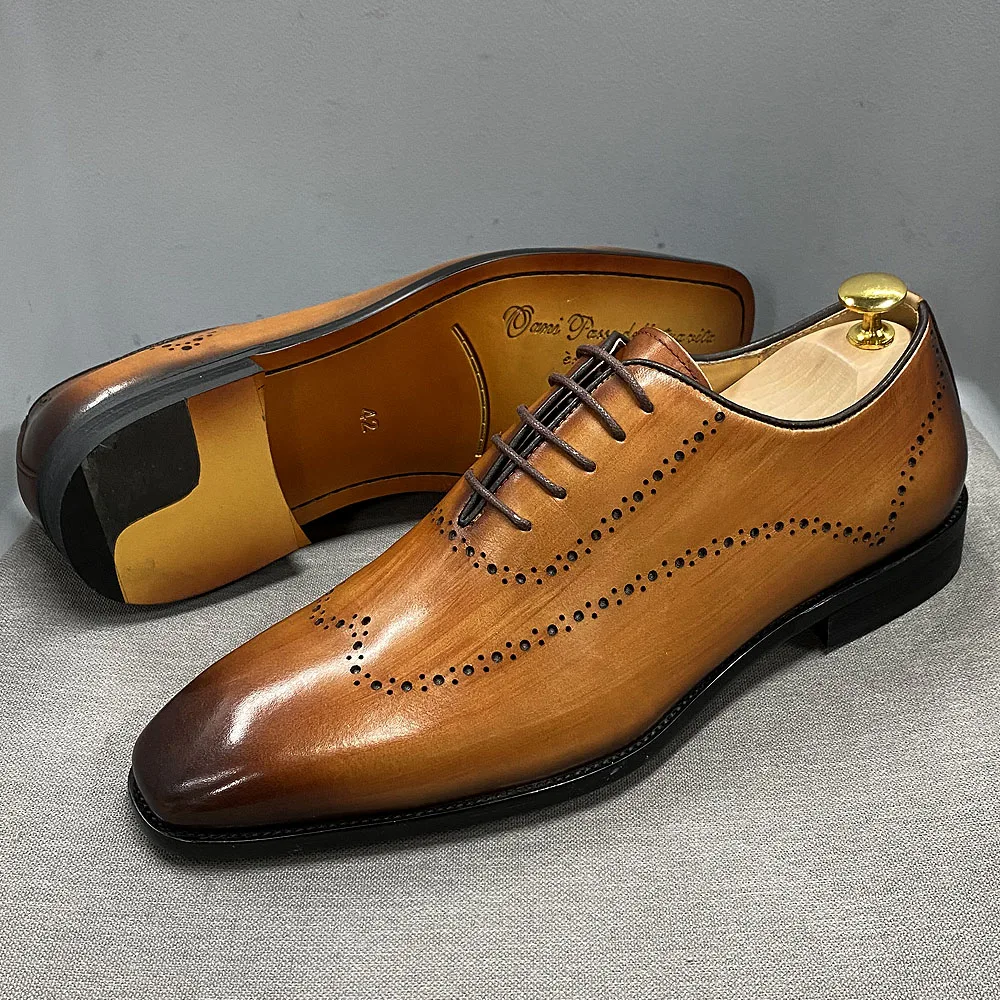The image features a pair of meticulously crafted brown shoes, positioned thoughtfully next to each other. One shoe displays its left profile, showcasing its sleek design, while the other shoe is laid on its back, revealing the intricate details of its sole. These shoes exude craftsmanship, with delicate, relatively thin shoelaces that are subtly integrated into the shoe's upper, concealing the knot. The attention to detail suggests the handiwork of a skilled shoemaker rather than mass production, characterized by the artistic elements and precision typically absent in off-the-shelf brands like Nike or Adidas.